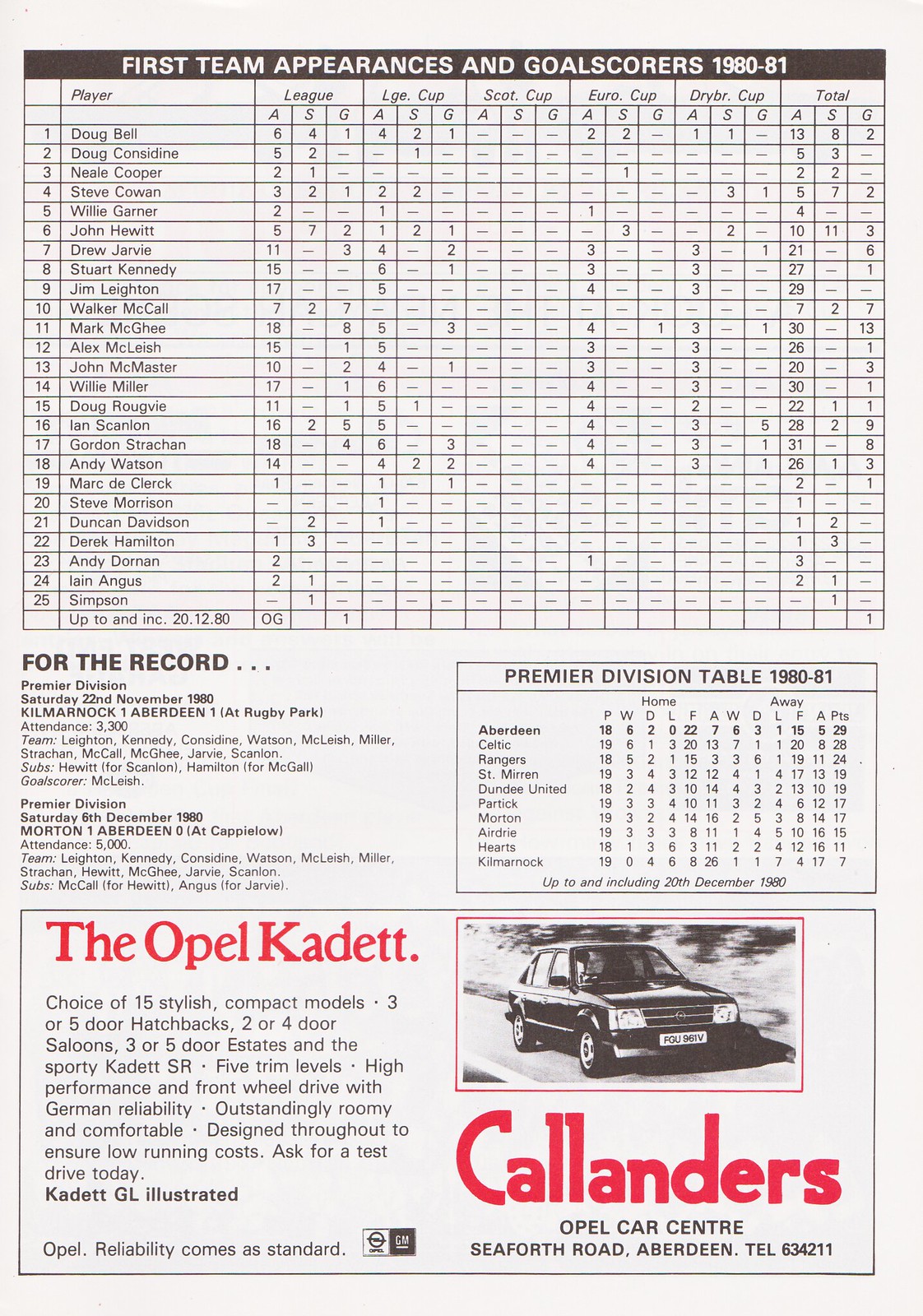The image depicts a detailed page from an old publication, possibly a sports program or magazine, divided into three distinct sections. At the top, there's a title reading "First Team Appearances and Goal Scores 1980 to 1981", accompanied by a comprehensive table listing 25 football players. The table includes detailed statistics for each player across different competitions: League, League Cup, Scottish Cup (Scott Cup), European Cup (Euro Cup), Drybrough Cup (DRYBR Cup), and totals. Below this, the second section, titled "For the Record," details notable Premier Division matches, specifically Kilmarnock vs Aberdeen on 22nd November 1980, which ended in a 1-1 draw with an attendance of 3,300, and Morton vs Aberdeen on 6th December 1980, which ended 1-0 in favor of Morton with an attendance of 5,000. This section also lists team members, substitutes, and goal scorers. To the right, there is a "Premier Division Table 1980 to 1981," showing the standings, points, goals, wins, and losses for different teams. The bottom section features an advertisement for the Opel Kadett, showcasing a black model with the number plate FGU 961 V. The ad highlights the choice of 15 stylish compact models, including 3 or 5-door hatchbacks, 2 or 4-door saloons, 3 or 5-door estates, and the sporty Kadett SR. It includes a note that the cars are available at Calendars, Opel Car Center, Seaford Road, Aberdeen, with a contact telephone number 634211.